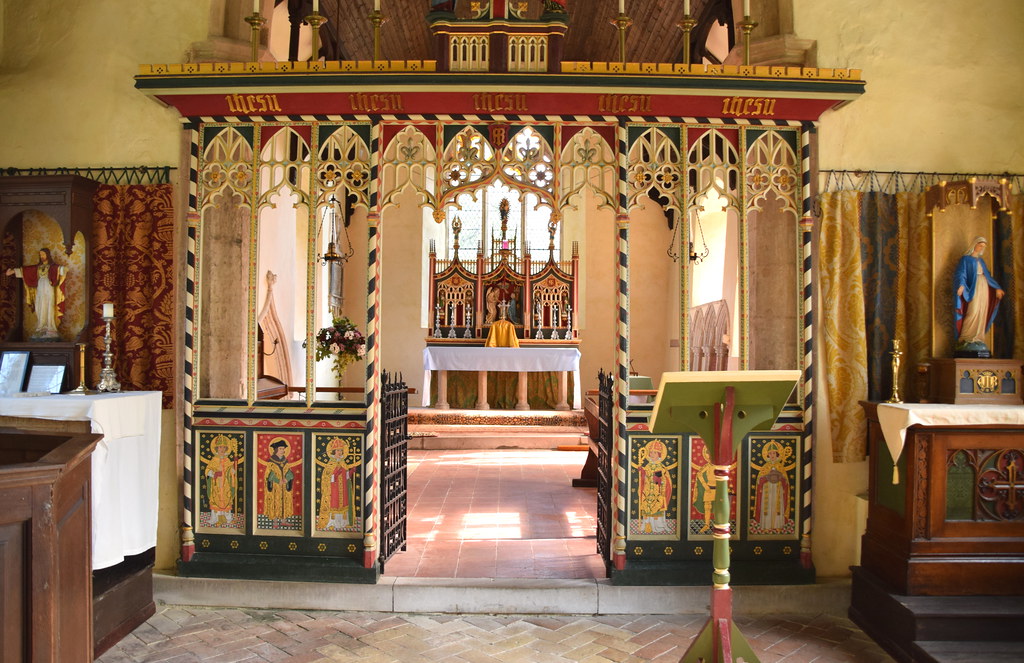The image captures the intricate interior of a historic church, adorned with vivid colors and religious decor. The stone flooring leads to a green and red pedestal on the right, likely used for reading scripture. This stand is situated in front of an ornate entryway that resembles an amusement park gate but features four posts with religious figures painted on them. The gate itself is waist-high and open, revealing a richly decorated backdrop with a triptych—the central panel depicting a cross on a special platform. To the right of the entryway, there's an inlet showcasing a statue of the Virgin Mary in a blue cloak, while to the left, a statue of Jesus in a red robe stands with his arms outstretched. A small altar in front of Jesus includes candles and pamphlets. Overhead, Latin inscriptions line the upper walls. Towards the back, more religious imagery and a large table are visible, completing the ornate and sacred atmosphere of the church.